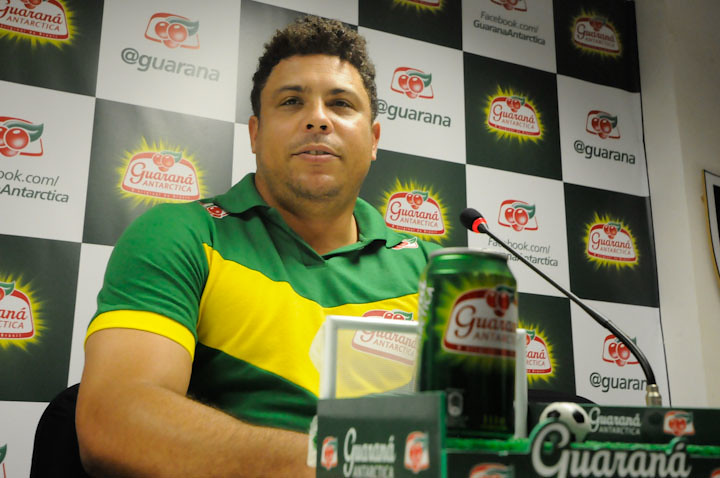In this detailed image, a tanned, curly brown-haired soccer player is seated behind a speaking table at what appears to be a post-game press conference. He is dressed in a green polo shirt with a yellow stripe, bearing the logo "Guarana, Antarctica." In front of him, arranged on a display podium that also features the word "Guarana," are a green can of the Walrodna drink and a small soccer ball. He also has a microphone aimed at him, ready for the interview. The backdrop behind him is a black-and-white checkered banner prominently displaying the Guarana logo, suggesting that the drink is a main sponsor. The setting and product placements indicate a promotional event following a game, hinting that he might have been the VIP player of the match.